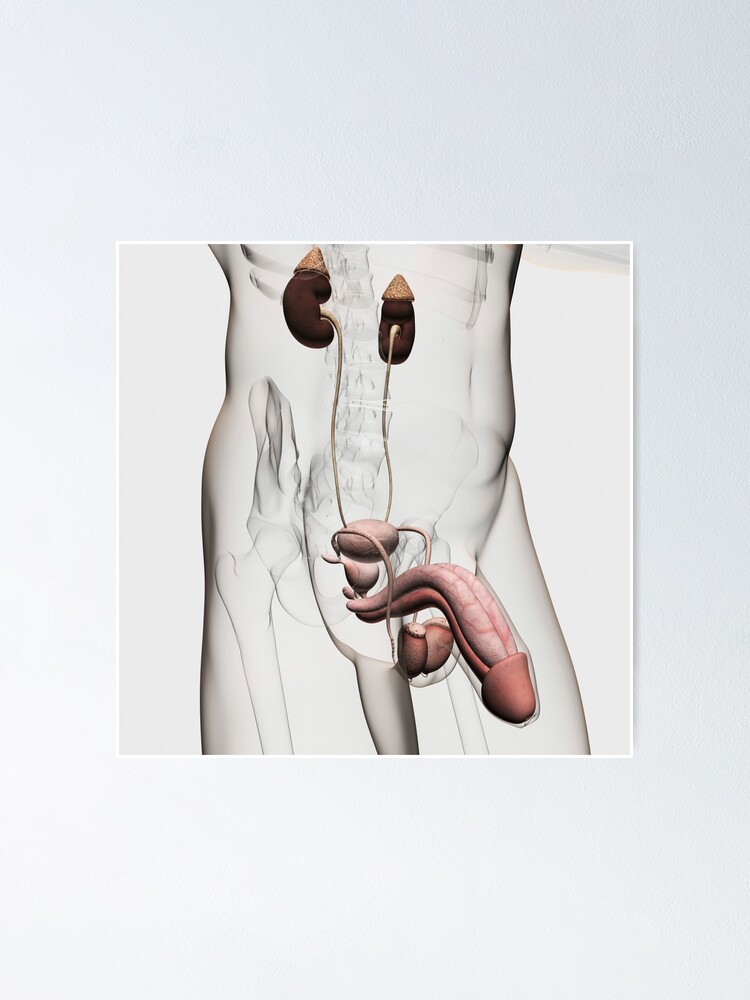The image is a detailed line drawing from a medical textbook, depicting the male torso from just below the chest to the mid-thigh region. This anatomical diagram highlights the internal organs and skeletal structure with vivid specificity. The spine, pelvis, and femurs are clearly outlined, with the entire body appearing semi-transparent to reveal the internal features. Central to the illustration are the kidneys, which are colored in a darker pink or brown hue and topped with tan-colored adrenal glands. These kidneys connect via winding cords to the urinary bladder, which is depicted as two spherical shapes stacked atop each other. Extending from the bladder is the male genital system, fully exposed to show the penis and testes. The internal structure of the testes is detailed, resembling brown nuts, while the spongy tissue inside the penis is also visible. The overall image is enclosed within a square, set against a larger white page.